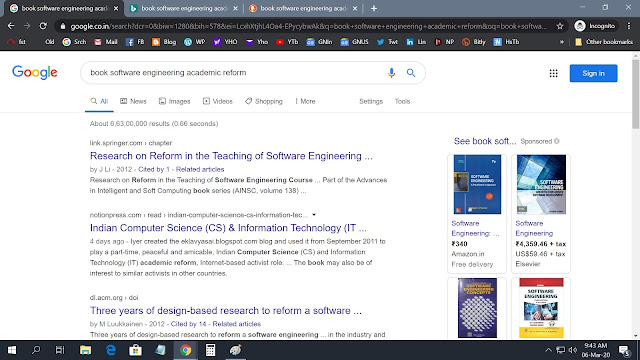The image shows a computer screen displaying the results of a saved search related to academic reform in the field of software engineering. The search appears to focus on the reform of teaching methods in software engineering, specifically within Indian computer science and information technology education. The top three search results listed include articles and research papers, with titles such as "Research on Reform in the Teaching of Software Engineering in Indian Computer Science and Information Technology" and "Three Years of Design-Based Research to Reform Software...". These titles hint at ongoing studies and efforts to improve the pedagogical approaches within this discipline.

On the right side of the screen, four books are displayed, presumably due to the search term "book." The first two book titles are clearly visible: "Software Engineering" and "Software Engineering," while the titles of the remaining two books are cut off at the bottom of the screen, making them unreadable.

The computer screen shows a timestamp of 9:41 a.m., and the system is running the Windows operating system.